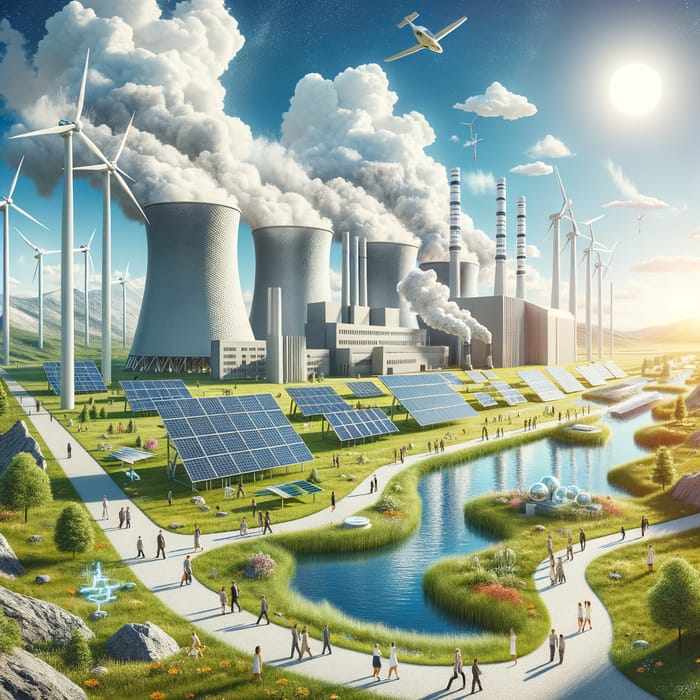This is a detailed, computer-generated image depicting a sustainable energy landscape. In the background, there is a power plant with four large, cylindrical smokestacks emitting thick, fluffy white smoke that drifts leftward. The sky is a deep blue, adorned with dispersed white clouds and featuring a white airplane flying overhead. The bright, glowing sun is positioned in the upper right corner of the image.

On either side of the smokestacks, tall wind turbines are visible, harnessing wind energy. The foreground showcases a lush, green area populated with various colored plants and dotted with rocks and boulders. A series of solar panels, prominently positioned under the smokestacks, are absorbing sunlight. These panels vary in size, with some divided into a six-by-four grid, while others are only two squares long.

A well-trodden sidewalk winds through the greenery, encircling a blue pond or lake. This path is frequented by several groups of people, walking or sitting on the grass, enjoying the serene environment. The image is further enriched with the presence of bulbous plant structures near the water. In the far distance, a mountain range completes the idyllic, renewable energy-focused scene.